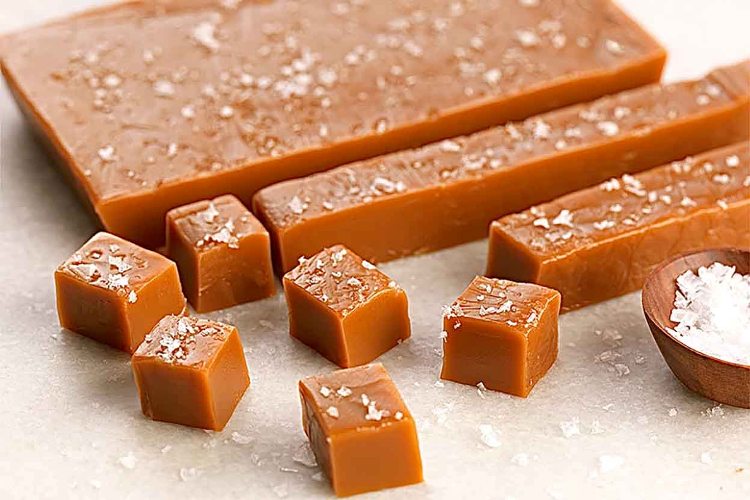A professionally taken image showcases a rich brown slab of caramel candy meticulously sliced and arranged on a white surface. In the foreground, the caramel is divided into six small cubes and two longer slices, all intricately decorated with large, white salt crystals. The caramel originated from a larger rectangular piece, which serves as a blurred backdrop in the image. To the right, there is a small wooden bowl filled with coarse salt, which is also lightly sprinkled around the table, adding to the overall texture and appeal. The entire scene, set on a pristine white table, highlights the contrast between the deep caramel and the glistening salt, making it an inviting, appetizing display.